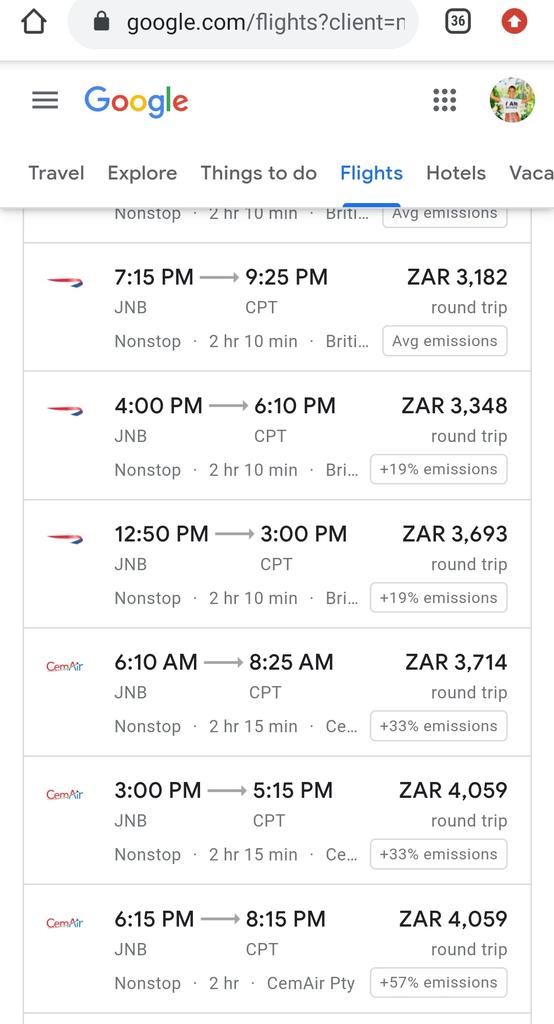A cropped image of a cell phone screen displays a web browser open to "google.com/flights." The URL includes a parameter that begins with "client=" and appears to be followed by a clipped-off character, possibly an "N." Notably, the user has an overwhelming 36 tabs open.

Below the URL bar, the header showcases the familiar Google logo, a hamburger menu icon for additional options, a 3x3 grid of dots likely for changing the display layout, and a circular avatar that is indistinguishable. The navigation tabs visible under the Google header include "Travel," "Explore," "Things to do," "Flights," "Hotels," and "Vacay" (short for "Vacation"). The "Flights" tab is currently highlighted.

The main content area lists flights departing from JNB (Johannesburg, South Africa) to CPT (Cape Town, South Africa), a journey of approximately two hours. Each entry on the right side shows the fare in "ZAR" (South African Rand) followed by a four-digit number separated by a comma, denoting the price with a thousand separator.

Despite the cluttered setup and some ambiguous elements, the image clearly focuses on searching for flights through Google's flight service.